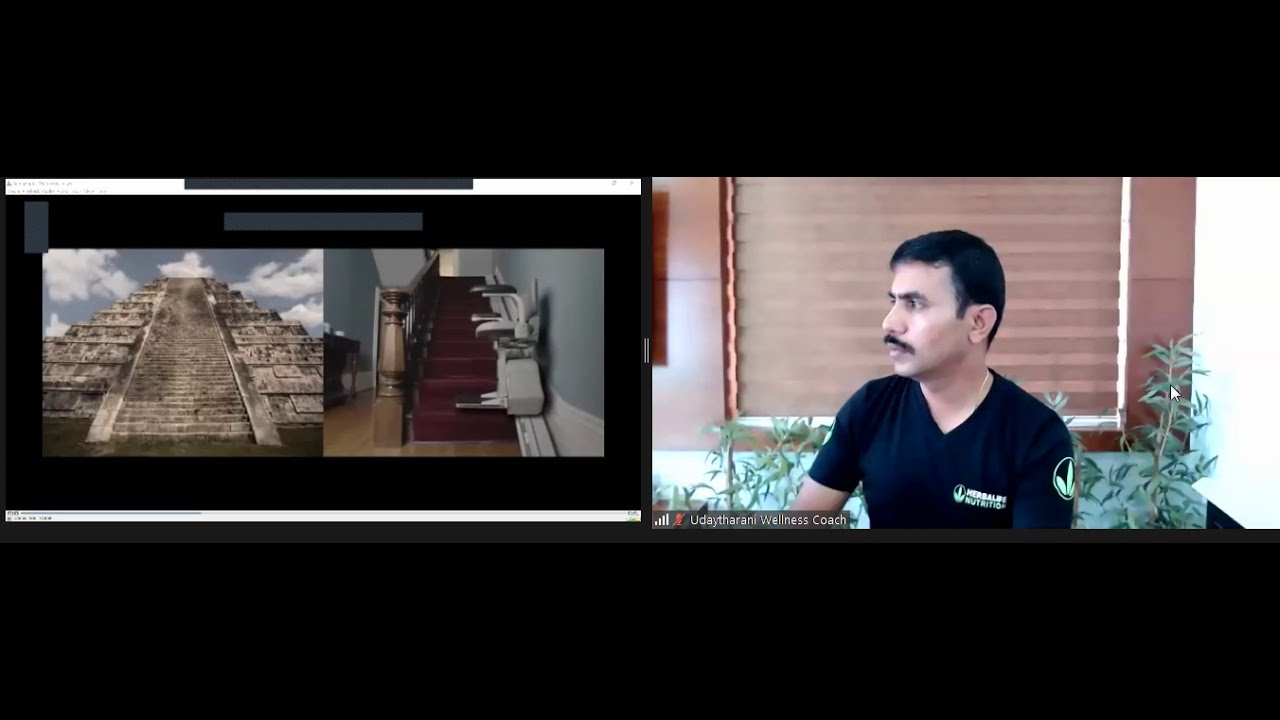The image shows a man with short black hair and a black mustache, wearing a black v-neck t-shirt with a white print that resembles a three-leaf plant. He is seated in a chair, possibly looking at a laptop or computer screen. Behind him, there's a window with a blind and a brown wall adorned with some plants. The overall scene is framed by black borders at the top and bottom, taking up a significant portion of the image.

On the left side of the screen, the monitor displays an image of an ancient Mayan pyramid with a blue sky and white clouds above it. On the right side, the screen shows the interior of a house, featuring stairs with red steps and a wooden railing. Additionally, a stair climber chair for disabled individuals can be seen ascending the stairs. The walls in this interior space are painted blue. The combination of these elements provides a detailed snapshot of a man engrossed in his activity, possibly reacting to the visuals on his screen, with diverse settings captured within the monitor.